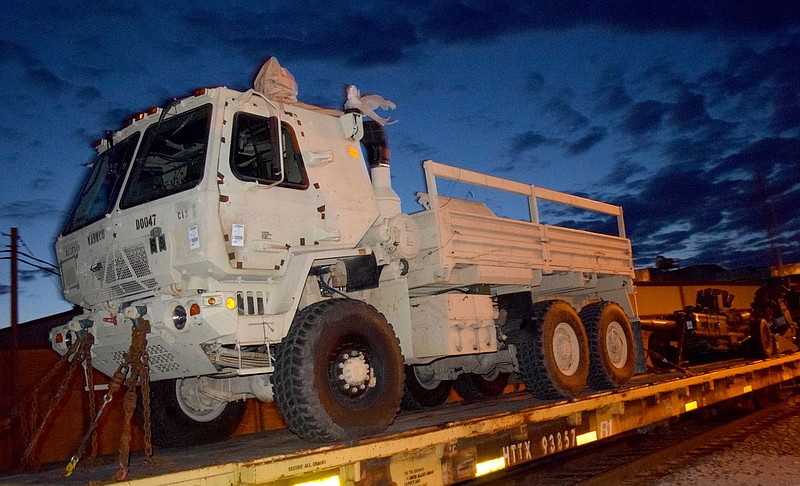This image features a light gray, six-wheel military-style vehicle secured on a flatbed trailer under twilight or early morning light. The vehicle has three large tires on each side and a distinct ride-over cab design with two sizeable front windows and additional large windows on either side. The open bed, lined with a side rail, appears to be designed to accommodate personnel, perhaps with benches inside and a flip-down back gate. The vehicle is chained down by two binders in the front, and a noticeable towing apparatus, potentially for a .50 caliber gun or similar low-profile equipment, is attached to the back bumper. The background includes a faded white horizon, transitioning to blue with dark clouds in the upper right. Below, a gravel surface is faintly visible. The side of the flatbed is marked with the code H2TX93857. The overall scene is cast in dim light with additional illumination likely from artificial sources, highlighting the vehicle's worn tires and rugged design.